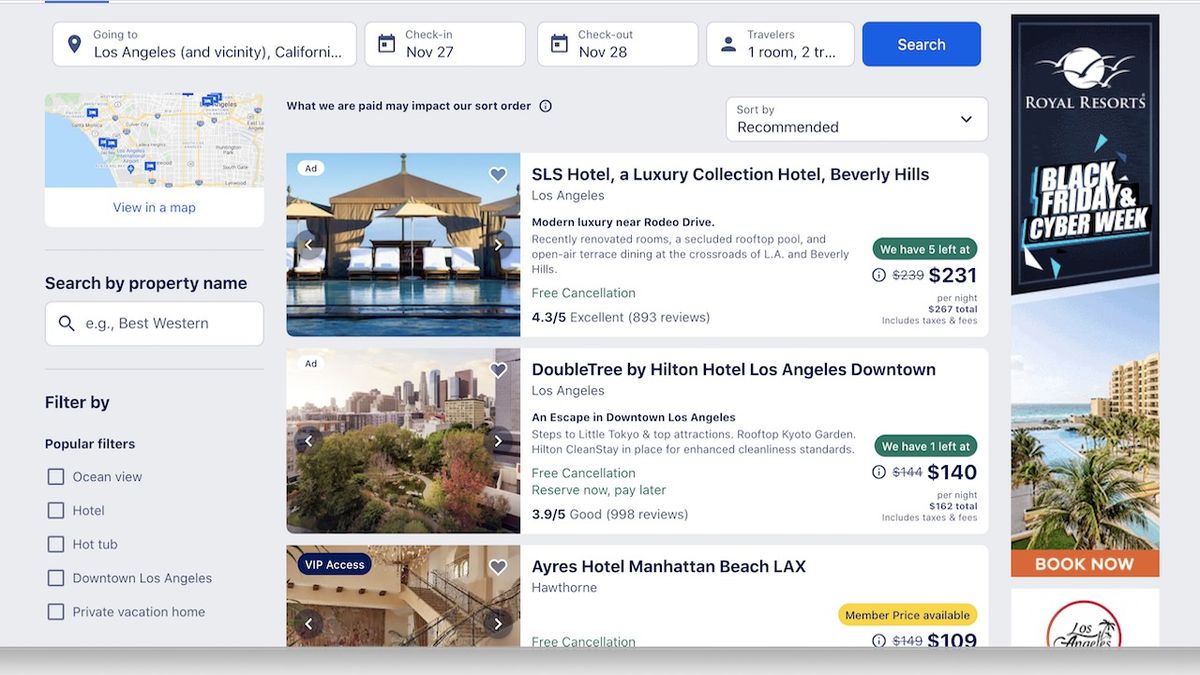The screen capture showcases a webpage displaying various hotel options in the Los Angeles area on a desktop computer. At the top of the screen, there are five buttons arranged side by side. Notably, the fifth button from the left is a blue search button. At the top left corner, there is a button labeled "Going to Los Angeles and vicinity, California." 

Beneath these buttons, a map of the California area is prominently displayed. Moving to the middle of the image, there are three pictures of different hotels, arranged vertically. The top image is accompanied by the text "SLS Hotel, a Luxury Collection Hotel, Beverly Hills, Los Angeles" beside it. To the right of this image, a green button is visible, with the price $231 listed in black text underneath it. 

Below the SLS Hotel image, two additional hotel options are displayed, each accompanied by their respective images and prices on the right side.